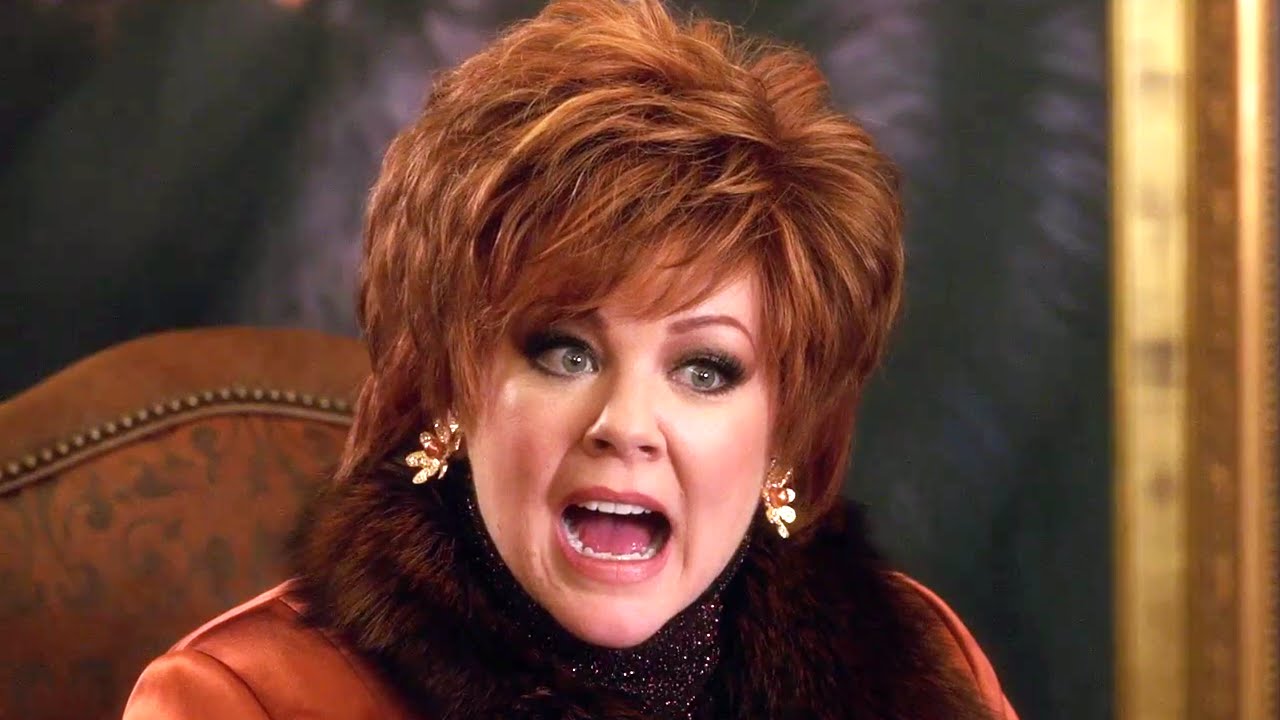This image features Melissa McCarthy, seemingly dressed in character for a role. She is seated in a brown upholstered chair decorated with a darker brown floral print and adorned with brass tacks around the top. Melissa sports a red bob haircut that falls over her forehead and above her ears, styled in a bouffant manner. She wears an orange velvet jacket with a brown fur collar, complemented by large gold earrings. Around her neck is a black and white speckled scarf. Her eyes are accentuated with dark makeup, and her mouth is open, giving the impression that she is yelling. The background behind her is predominantly dark and out of focus, with a gold frame running along the right side, suggesting part of a wall or a decorative element.